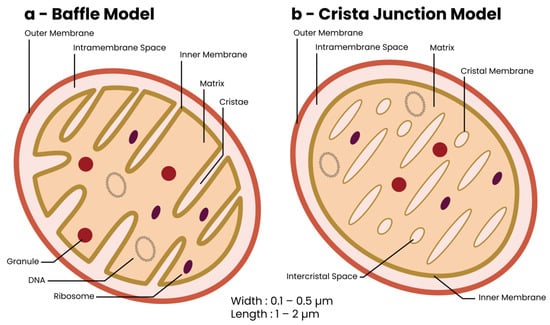This detailed biological diagram, likely from a college textbook, illustrates two mitochondria models: the Baffle model (A) and the Crista junction model (B). Both models are depicted in a sliced view to expose the inner and outer membranes, the intramembrane spaces, and the matrix. The diagram highlights membrane widths, measured in micron units (0.1 to 0.5 microns), and mitochondria lengths ranging from 1 to 2 microns. Model A, the Baffle model, features an intricately folded inner membrane resembling a "monster plant," dotted with granules (red), DNA (purple), and ribosomes. In contrast, Model B, the Crista junction model, showcases a crystalline inner membrane with distinct crista spaces but lacks labels for granules, DNA, and ribosomes. The membranes are depicted in shades of flesh, rust, and pink, with black lettering for labels, indicating its educational purpose within the textbook's context.